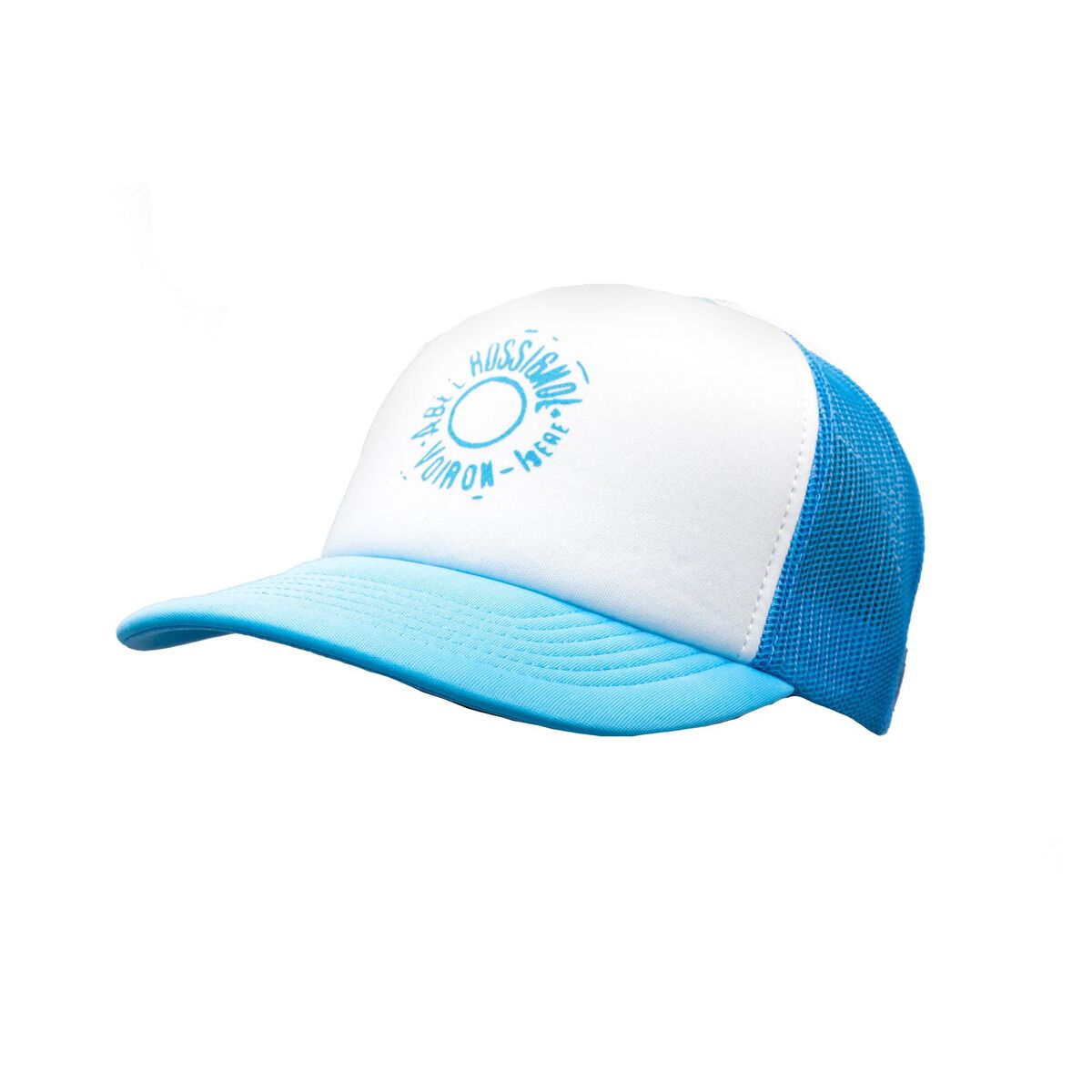The image features a blue and white baseball cap prominently displayed against a completely white background. The cap has a white front panel adorned with illegible text arranged around a light blue circle. The text appears to read "H-O-S-S-I-G-N-O-L" with "Boiron" and "HERE" included, though the exact wording is unclear. The bill of the cap is light blue, matching the blue mesh back that resembles plastic webbing. This stock image, oriented slightly to the left, showcases a traditional five-panel design with five U-shaped stitches connecting the bill to the hat.